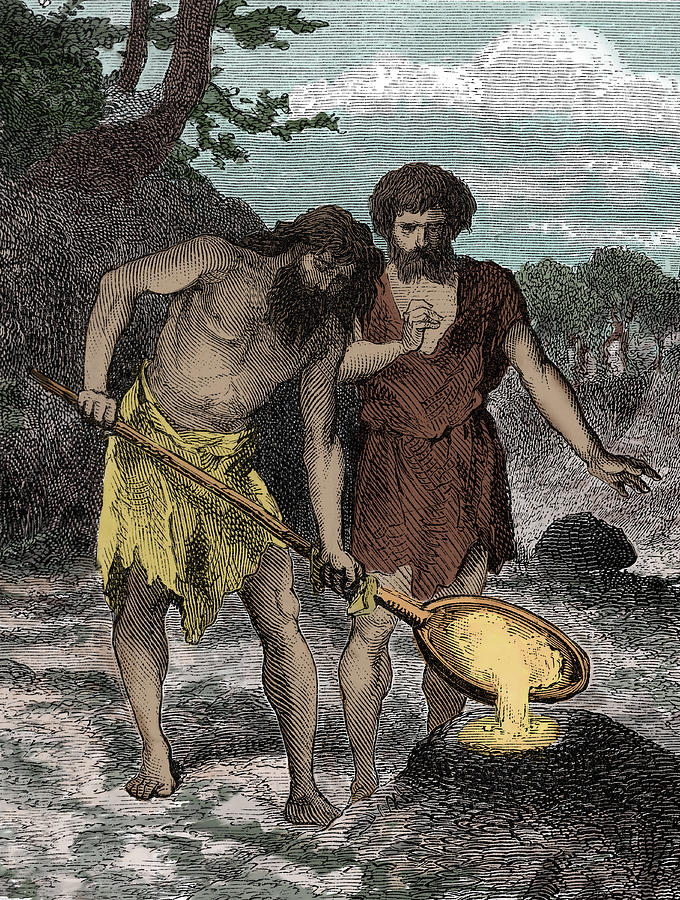The image is a detailed etching with coloring, depicting a scene from what appears to be the Bronze Age or medieval times. It focuses on two bearded men with long hair working in a field under a light blue sky dotted with clouds. The man on the left is shirtless and wears a yellow loincloth. He is holding a large wooden spoon filled with a yellow substance, which he is pouring into a hole or a mound of rocks or dirt in the foreground. The man on the right wears a light brown, ragged tunic that reaches above his knees. Both men are engaged in what seems to be a metal-smelting process. In the background, dark trees frame the scene, contributing to the historical and rustic atmosphere.